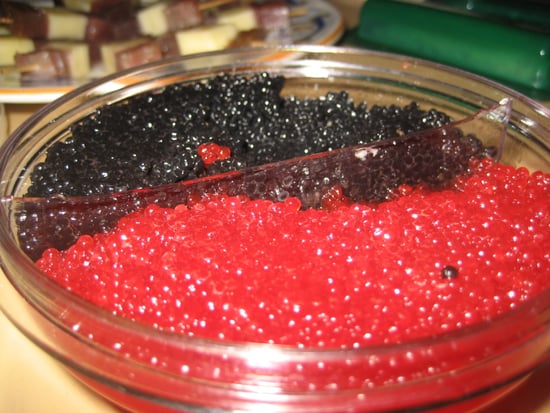The image shows a circular, see-through glass dish with a built-in divider creating two halves. On the lower right, the dish holds red caviar, and on the upper left, it contains black caviar. The arrangement mimics a yin-yang symbol, with a single piece of black caviar in the red section and a few red caviar pieces in the black section. The dish is set on a light brown counter. In the distant background, there is a blurry platter, possibly containing cheese cubes, and a green cylinder lies on its side in the top right corner.